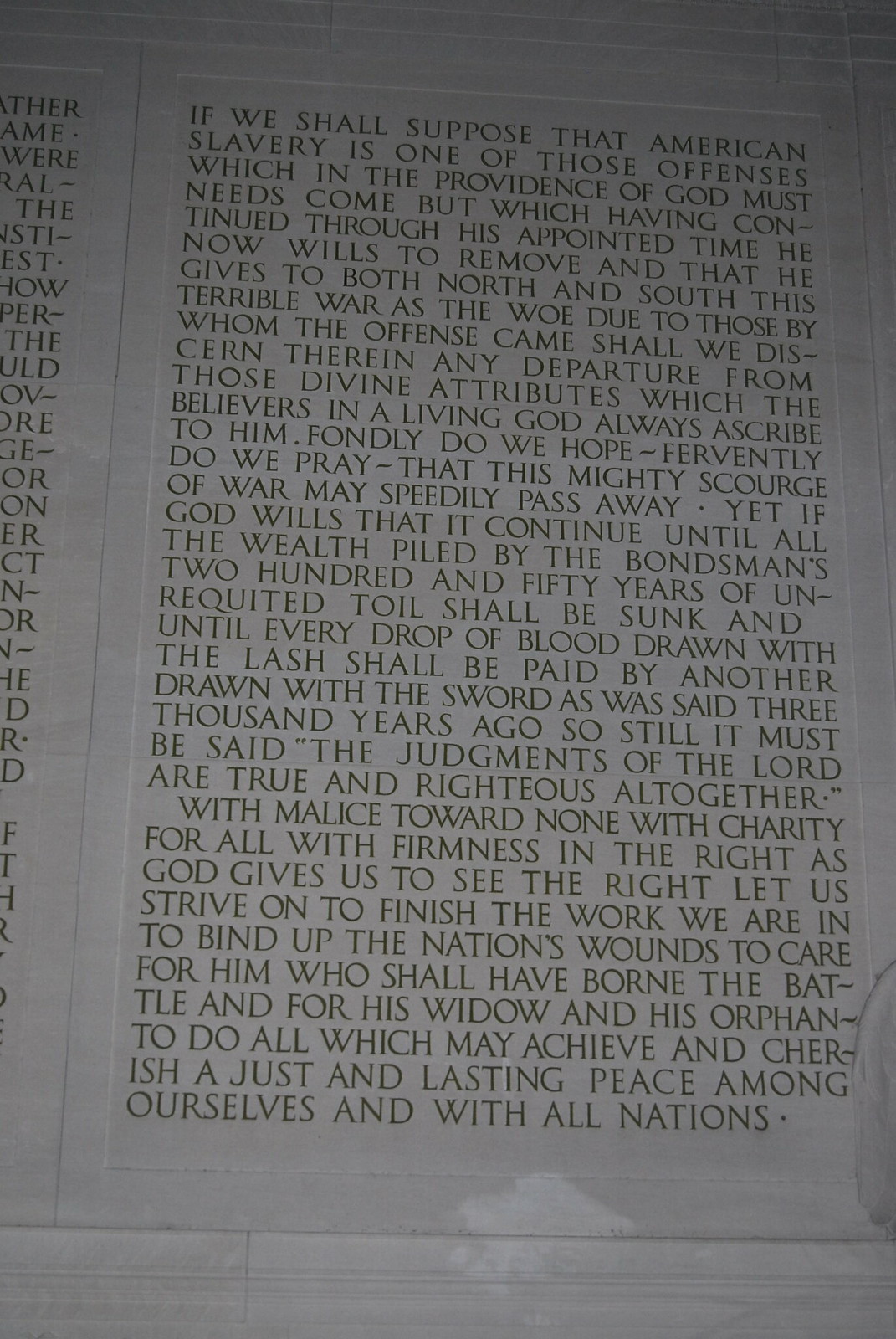The image showcases a large, white-gray stone slab with black engraved text that appears sophisticated and enduring, possibly part of a stately building or monument. The passage reflects on American slavery and the Civil War, framed as events within the providence of God, emphasizing that the war serves as divine retribution for the offense of slavery. The text likely continues a famous quote, perhaps from a prayer or a historical speech, urging hope and prayer for the end of the conflict and advocating for a just and lasting peace. The engraving reads: "If we shall suppose that American slavery is one of those offenses which in the providence of God must needs come, but which having continued through his appointed time, he now wills to remove, and that he gives to both North and South this terrible war as the woe due to those by whom the offense came, shall we discern therein any departure from those divine attributes which the believers in a living God always ascribe to him, fondly do we hope, fervently do we pray, that this mighty scourge of war may speedily pass away, yet if God wills that it continue until all the wealth piled by the bondsman's two hundred and fifty years of unrequited toil shall be sunk and until every drop of blood drawn with the lash shall be paid by another drawn with the sword, as was said three thousand years ago, so still it must be said, 'The judgments of the Lord are true and righteous altogether.' With malice towards none, with charity for all, with firmness in the right as God gives us to see the right, let us strive on to finish the work we are in, to bind up the nation's wounds, to care for him who shall have borne the battle and for his widow and his orphan, to do all which may achieve and cherish a just and lasting peace among ourselves and with all nations." On the left edge of the image, another column of text is partially visible, suggesting the presence of more engraved text on an adjacent stone.